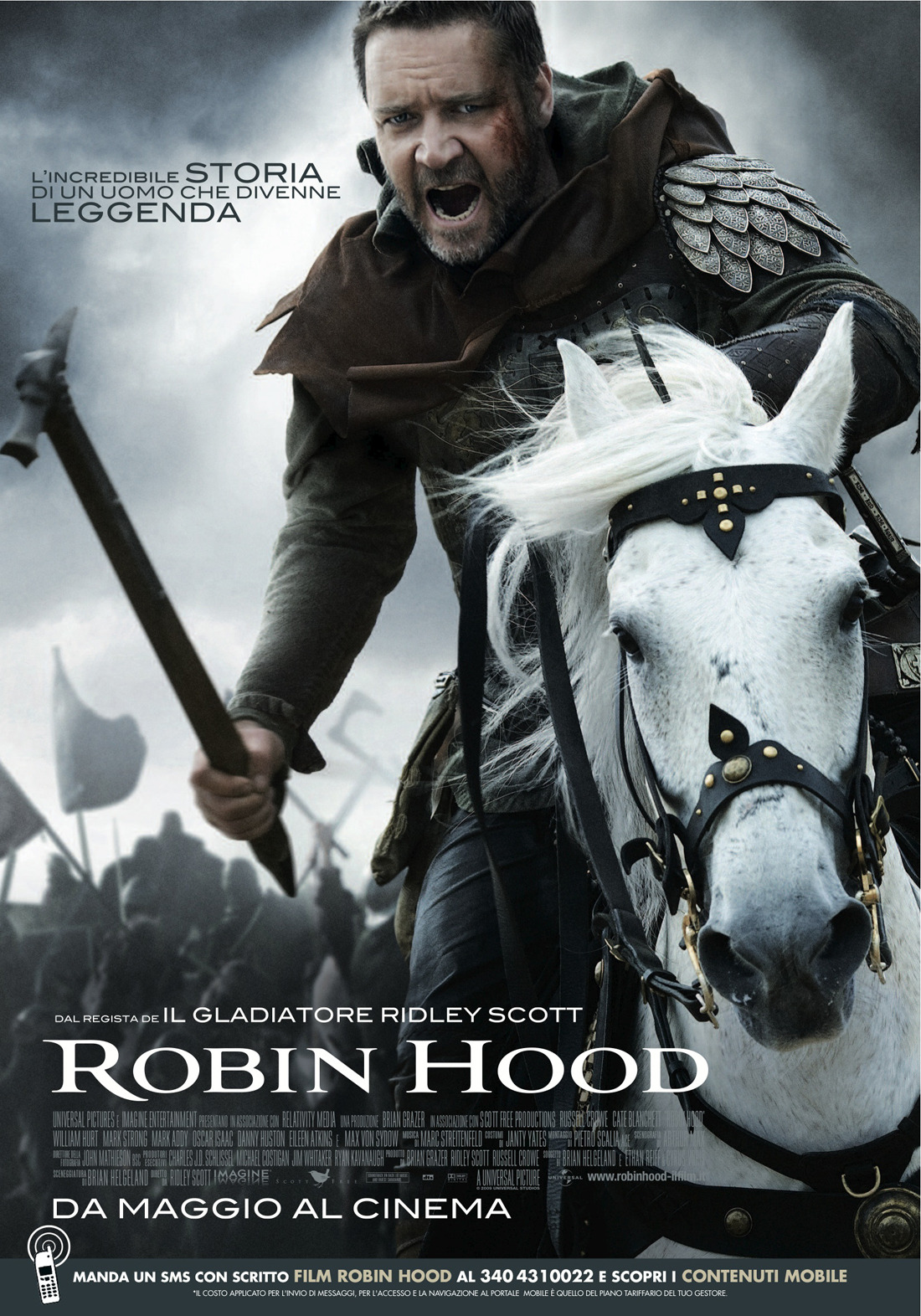This is an intricate movie poster for "Robin Hood," directed by Ridley Scott and starring Russell Crowe, who is prominently featured at the center. The vertically-oriented poster showcases Crowe mounted on a white horse adorned with a black leather harness with gold metal parts. Crowe, wielding a war hammer in his right hand and wearing feather-like shoulder armor, has a fierce expression with an open mouth and blood on the side of his face. He is clothed in traditional period attire.

The backdrop of the poster is a stormy, overcast sky with white and gray smoke, indicating a medieval battle with blurred soldiers and flags, creating a chaotic battlefield scene. Text on the poster includes large white uppercase lettering of the movie title "Robin Hood" at the bottom, while additional information in white and black text, including the phrases "Dal Regista de Il Gladiatore Ridley Scott" and "Dal Maggio al Cinema," are present, emphasizing its Italian release. The poster is distinctly muted, primarily using black, white, and gray tones, reinforcing the dramatic and intense atmosphere of the film’s setting.